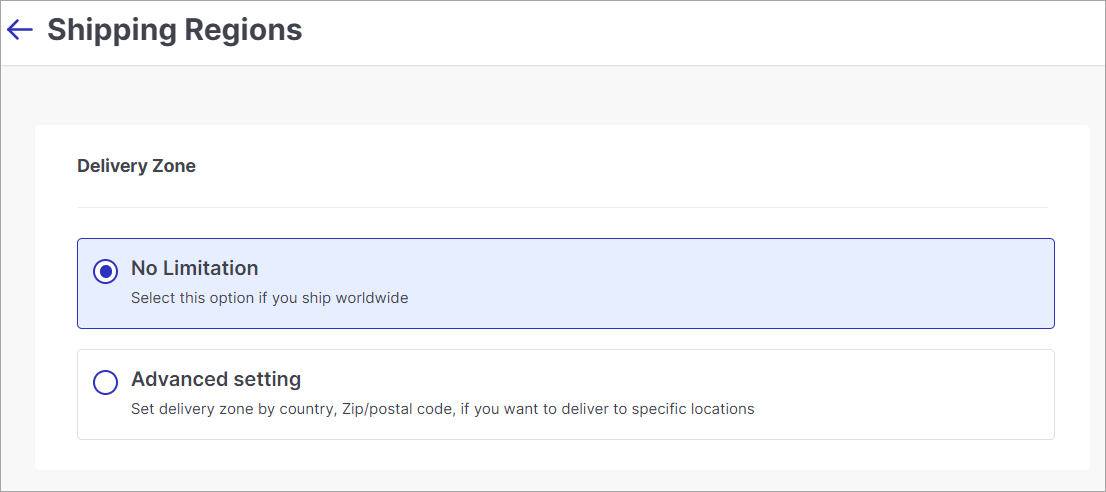The image is a screenshot of a device screen displaying a user interface for setting shipping preferences. At the top of the screen, the title "Shipping Regions" is prominently displayed. On the left side of this title, there is a purple arrow icon pointing to the left. The background of the interface is primarily light gray.

Below the title, there is a section labeled "Delivery Zone" which indicates the current setting of "No Limitation." This section is encased in a bluish box outlined with a light purple line, highlighting its selection. Within the "No Limitation" option, there is a purple circle inside a white circle, signifying that this option is currently selected. Next to this, there is a description stating, "Select this option if you ship worldwide."

Further down, there is another option labeled "Advanced Setting," which is not selected. This option features additional instructions: "Set Delivery Zone by Country, Zip/Postal Code, if you want to deliver to specific locations." The white interior box that contains these options contrasts with the light gray background, and a subtle border of colors delineates different sections of the interface. The bottom right corner of the screen exhibits this transition clearly, with alternating gray and white hues.